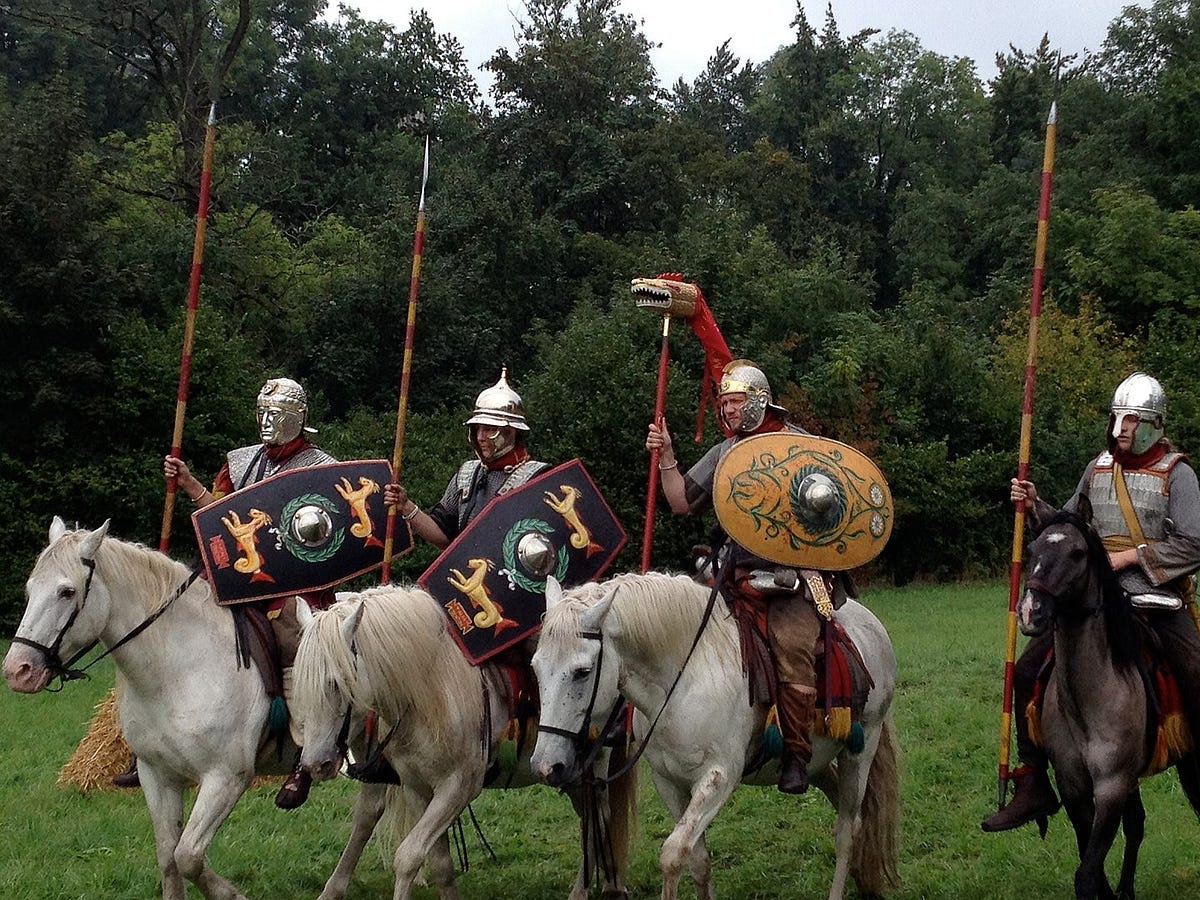A scene captured from a historical reenactment portrays four knights in a woodland setting, full of green and yellow-leafed trees with a sky of white and blue hues. The knights, clad in a variety of elaborate armor, are mounted on horses: the three on the left ride white steeds while the knight on the far right is astride a brown horse. The knight on the far left wears a full-face silver mask and a red and yellow outfit, carrying a red and yellow pole with a silver tip. His shield is oval-shaped, brown with floral decorations. The next knight sports a simple silver helmet, a red-lined shield, and holds a spear. The third rider dons a traditional Roman helmet and holds a shield decorated with green leaves and a silver center, his red pole featuring a dragon's face. The final knight, on the brown horse, wears a medieval helmet, partial facial cover, and full frontal silver armor with yellow straps. He holds a red and yellow striped pole with a silver tip. The grass underfoot is vividly green, with a haystack visible near the first horse.